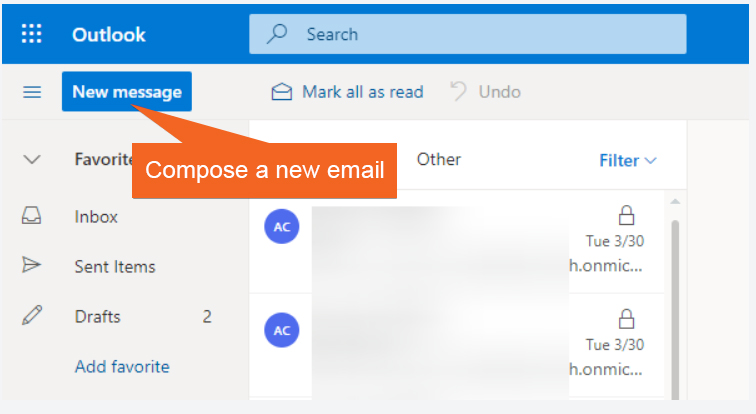The image is a screenshot of a desktop or mobile Outlook email interface, highlighting various interface elements. 

At the top, the "New Message" tab is prominently highlighted in blue, accompanied by a large orange pointer emphasizing the option to "Compose a new email." 

On the left, there's a vertical navigation pane featuring several tabs: "Favorites," "Inbox," "Sent Items," and "Drafts," which appear twice. Below these tabs, a blue "Add Favorite" button is visible.

Shifting to the middle-right, the uppermost part of the pane displays buttons labeled "Mark all as read" and "Undo." Below, the preview pane shows two emails from a sender identified by the initials "AC," marked with a blue circle. Although the exact subject lines are cut off, the emails are timestamped as Tuesday at 3:30 and contain partially visible headers with "H-O-N-M-I-C" and "H.O-N-M-I-C" respectively.

Above the preview pane, a search bar with a magnifying glass icon allows users to search through their emails. Just beside the "Outlook" label, there is an icon with six dots, presumably for accessing additional options.

Moreover, next to the "Inbox," "Sent Items," and "Drafts" tabs, small icons provide visual identifiers—a mail icon for the inbox, a sent mail icon for the sent items, and a pencil or pen icon for drafts. This detailed layout captures the essential elements of the Outlook interface as seen in the screenshot.